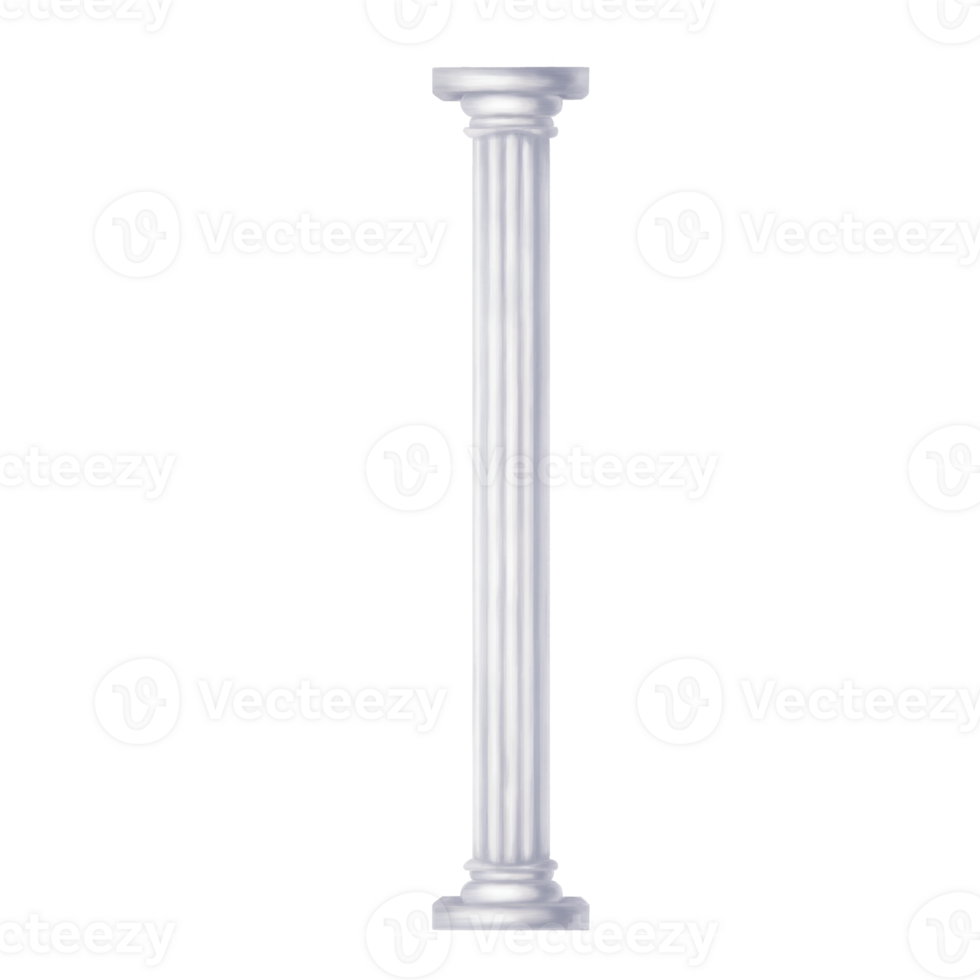This is a detailed black and white illustration of a Roman Doric column with a fluted design, centrally positioned on a plain white background. The column features a pedestal at the bottom and a squared top with flared, flat details. It incorporates a mix of rounded and squared surfaces. The image is extensively watermarked with the word "Vecteezy" (spelled V-E-C-T-E-E-Z-Y) alongside a stylized logo of a "V" within a circle. These watermarks are printed transparently and repeatedly across the image, indicating the stock photo origin. There are no people, animals, or additional text present in the image.